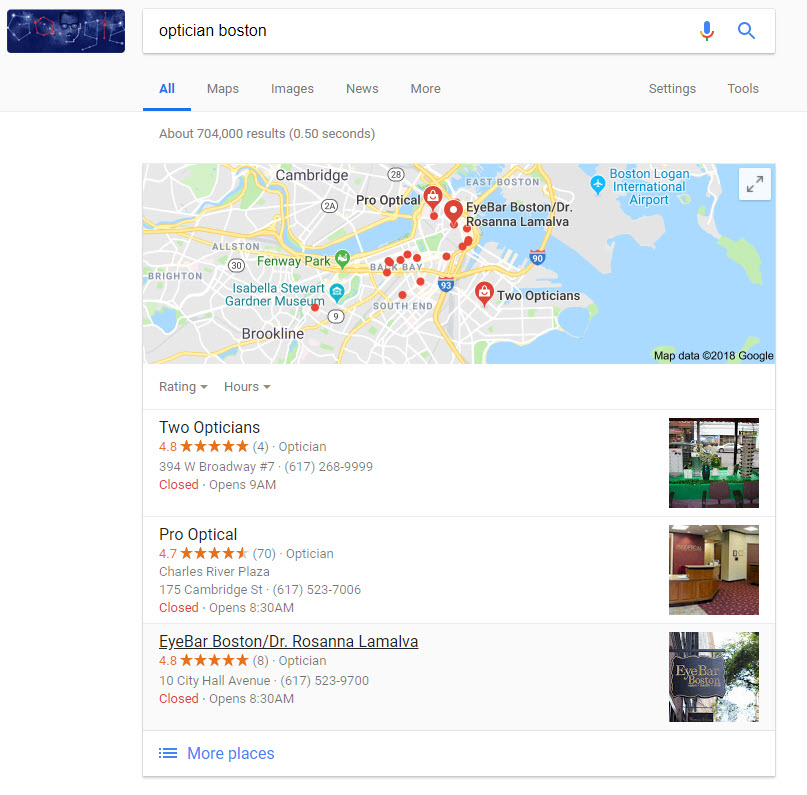Here's a refined and detailed caption for the described image:

The image is a screenshot from a Google search for "Optician Boston." The Google logo in the top-left corner presents an eerie transformation, featuring a night sky backdrop with stars connecting to form a zombie-like face, potentially depicting a scientist with eyeglasses. The search bar contains the query "Optician Boston," accompanied by the microphone icon and magnifying glass, while the interface elements "Maps," "Images," "News," "More," "Settings," and "Tools" are all displayed in gray. Below the search bar, it shows there are approximately 704,000 results found in just 0.50 seconds.

A map of the Boston area occupies the main portion of the screen, highlighted with multiple red markers—each representing optician locations. Three of these markers are adorned with shopping bag icons indicating special listings. Prominent landmarks such as Boston Logan International Airport, Isabella Stewart Gardner Museum, Brookline, Cambridge, Brighton, Allston, South End, East Boston, Back Bay, and Fenway Park are visible on the map.

Beneath the map, results for opticians are listed, each with relevant details:

1. **Optician** - 4.8 stars from 4 reviews, located at 394 West Broadway, number 7 (phone: 617-268-9999). The store is currently closed and will open at 9 a.m. The accompanying image appears to show the inside of the store, with eyeglasses on display racks, chairs in the foreground, and a clear view of the street through the front windows.

2. **Pro Optical** - 4.7 stars from 70 ratings, situated at Charles River Plaza, 175 Cambridge Street (phone: 617-523-7006). This location is currently closed and will open at 8:30 a.m. The image provided depicts the lobby area with maroon carpeting, maroon and yellow walls, and a wooden front desk.

3. **Ibar Boston/Dr. Rosanna LaMalva** - 4.8 stars from 8 reviews, located at 10 City Hall Avenue (phone: 617-523-9700). This establishment is also closed, opening at 8:30 a.m. The image shows an office space, though specific interior details are not provided.

At the bottom of the search results, there is a link in blue labeled "More places," accompanied by a hamburger menu icon, suggesting more options can be revealed.